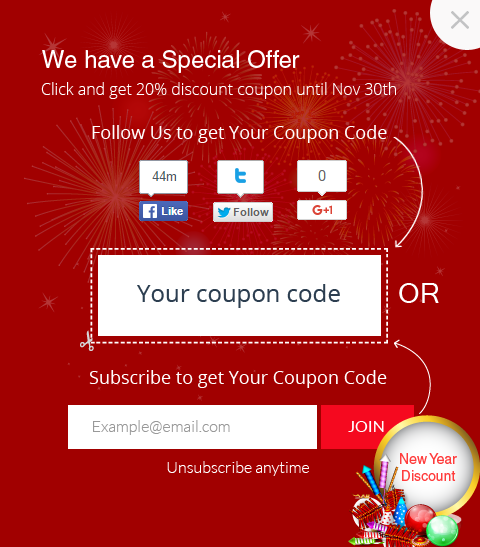The image depicts a promotional interface, likely on a website or app, with a visually appealing Christmas-themed background. The background is predominantly a dark, festive red, reminiscent of traditional Christmas ornaments. Embedded within this red expanse are starbursts and stars with four-pointed ends, interspersed with dots, all rendered in a slightly lighter shade of red, creating a subtle and cohesive design.

In the upper right corner, there is a gray "X" icon, suggesting the option to close or dismiss the promotional overlay. The primary text is displayed on the left side in white letters. At the top, there is a bold, large text stating, "We Have a Special Offer." Immediately underneath, in smaller text, it reads, "Click and get a 20% discount coupon until November 30th."

Beneath this, a slightly indented line of text instructs, "Follow us to get your coupon code," accompanied by a swooping arrow that curls towards the right and downwards, pointing to a horizontal rectangle in the middle of the page. This rectangle, framed by a dotted line, features a scissor icon in the lower left corner and the phrase "Your Coupon Code" centered within it.

To the right of the rectangular coupon code section, the word "Order" is printed. Below this, there is an invitation to "Subscribe to get your coupon code," along with a designated input box for entering an email address. Adjacent to this input field is a "Join" button, ready to facilitate the subscription process.